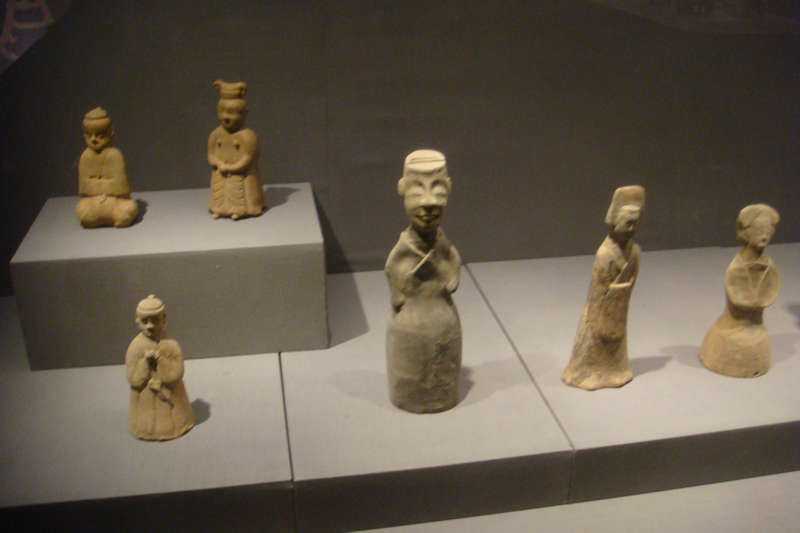This somewhat blurry photograph captures a display in a museum showcasing six small, clay figurines, all brownish in color. These artifacts, possibly originating from various ancient cultures in Asia, are arranged within a gray display case on a two-tiered platform. On the lower level, which seems to be crafted from segments of stone or brick, four statues are aligned. From left to right, the leftmost figure is a man kneeling in prayer, followed by a larger central statue of another kneeling man, and then a woman standing with her hands clasped in front of her. The rightmost two statues include the smallest figure in the formation.

Behind the leftmost figure on the lower level, there is a second taller rectangular base, also made of a similar stone or brick material. Atop this taller base, two more statues are placed: one depicting a woman in a long robe with a tall hat and another woman standing with a hat, a long dress, and her arms crossed in front of her chest. The detailed composition and careful arrangement of the figures highlight the cultural and artistic significance of these ancient artifacts.